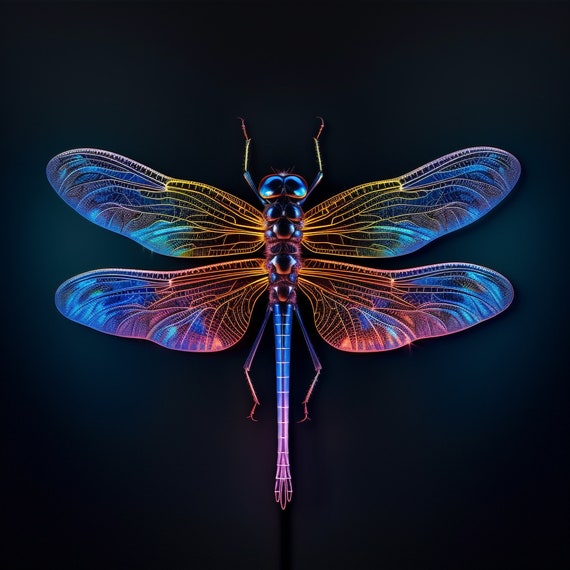This image presents a vividly colorful dragonfly, captured from a top-down view against a stark black background. The dragonfly's body is a striking array of neon and rainbow hues, with its tail glowing pink and blue, and its body radiating red. The four wings exhibit a translucent quality reminiscent of an x-ray, adorned with intricate veins that branch out like delicate leaves. The colors of the wings transition from yellow near the body to pink and blue at the edges, enhancing the ethereal glow against the dark backdrop. The overall appearance is almost surreal, resembling a cyberpunk or AI-generated art piece with its techno iridescence and vibrant palette of blue, yellow, orange, pink, turquoise, and purple. The glowing, thin lines create a mesmerizing, neon-like effect, making the dragonfly seem embellished or CGI-rendered, as it stands out intensely from its surroundings.